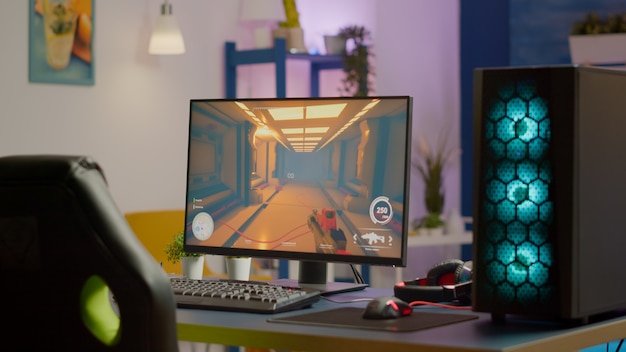This color photo captures an inviting and meticulously organized home office space that's clearly set up for gaming. Central to the image is a sleek, black gaming computer, which is illuminated with vibrant blue neon lights, adding a touch of futuristic flair. The monitor, positioned to the left of the PC, displays an intense first-person shooter game, clearly showing the player's perspective with a visible gun in hand. The desk is neatly arranged with essential gaming peripherals: a keyboard front and center, a red neon-lit gaming mouse to its right, and a pair of headphones lying nearby. Large, imposing speakers, also glowing blue, flank the setup, hinting at an immersive audio experience. The black leather desk chair faces the computer, ready for the next gaming session. The background features a tall bookshelf adorned with a planter on top, adding a touch of greenery. Warm lighting from a turned-on fixture casts a cozy glow over the space, while tasteful wall decor, including paintings, enhances the ambiance, suggesting a well-lived-in and cared-for home.